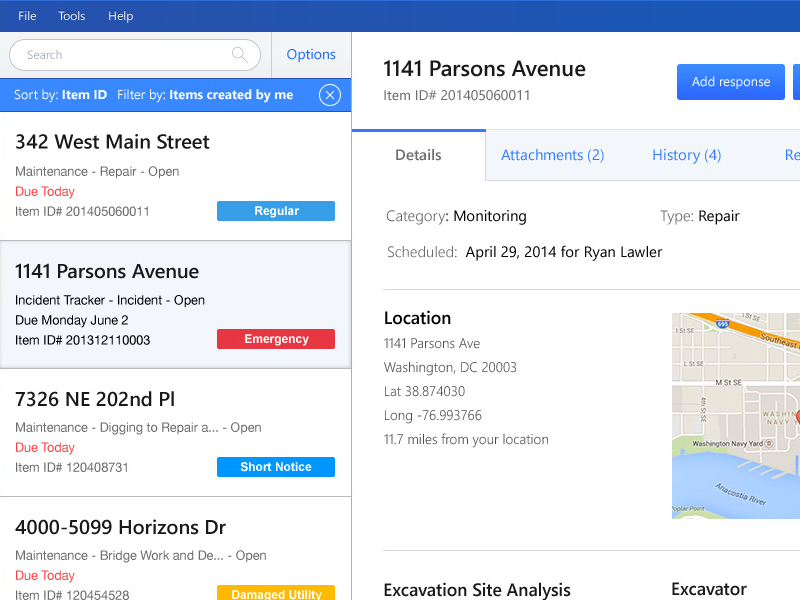The image appears to be a screenshot from an application designed for maintenance and repair personnel. The left side of the screen lists different addresses and their corresponding maintenance instances. The current entries displayed are:

1. **342 West Main Street**: A regular maintenance repair due today.
2. **1141 Parsons Avenue**: An emergency incident tracker indicating an open incident due by Monday, June 2nd.
3. **7326 Northeast 202nd Place**: A short notice maintenance digging request to repair an unspecified issue, with details cut off. This task is also due today.
4. **4099 Horizons Drive**: Maintenance work on a bridge, labeled as a damage utility issue, due today.

For the address **1141 Parsons Avenue**, which is currently selected for the emergency incident, the details tab is shown along with available tabs for attachments, history, and an additional tab that is cut off from view. The detail tab specifies an excavation site analysis, mentioning:

- **Excavator**: Ryan Lawler, scheduled for April 29th, 2014.
- **Category**: Monitoring.
- **Type**: Repair.
- **Location**: 1141 Parsons Avenue, Washington, D.C., 20003.
- **Coordinates**: 11.7 miles from the user’s current location.

This application is clearly intended to help maintenance and repair personnel track, manage, and access detailed information regarding current incidents and scheduled repairs before they head out to the respective sites.